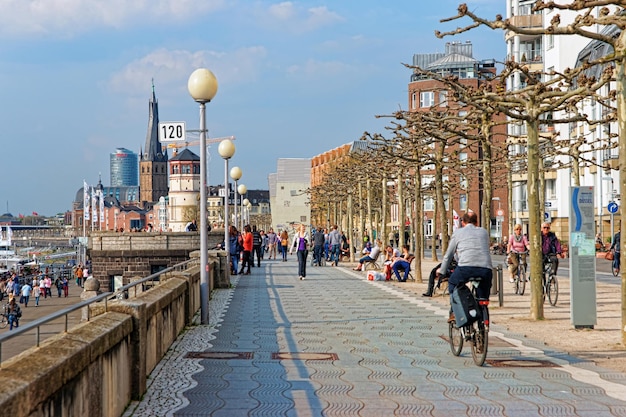The photograph depicts a bustling, modern European city, likely somewhere in Germany. Taken from a slightly elevated perspective along a scenic promenade, the image showcases a broad, walkable area paved with tiles featuring a wavy white line pattern. To the left of this pathway, a concrete guardrail overlooks a lower-level promenade filled with additional pedestrians. The right side of the promenade is lined with tall, woody trees and benches, providing a natural contrast to the urban environment. Spherical street lamps dot the left side of the pathway, adding a classic touch. A cyclist rides along a blue bike path that runs parallel to the promenade, heading into the distance. The cityscape in the background features a mix of residential and commercial buildings, including some notable church structures, all standing around four to five stories tall. The sky above is cloudy with large, fluffy clouds, suggesting a mild day typical of spring, with temperatures comfortable enough for people to wear light sweaters.